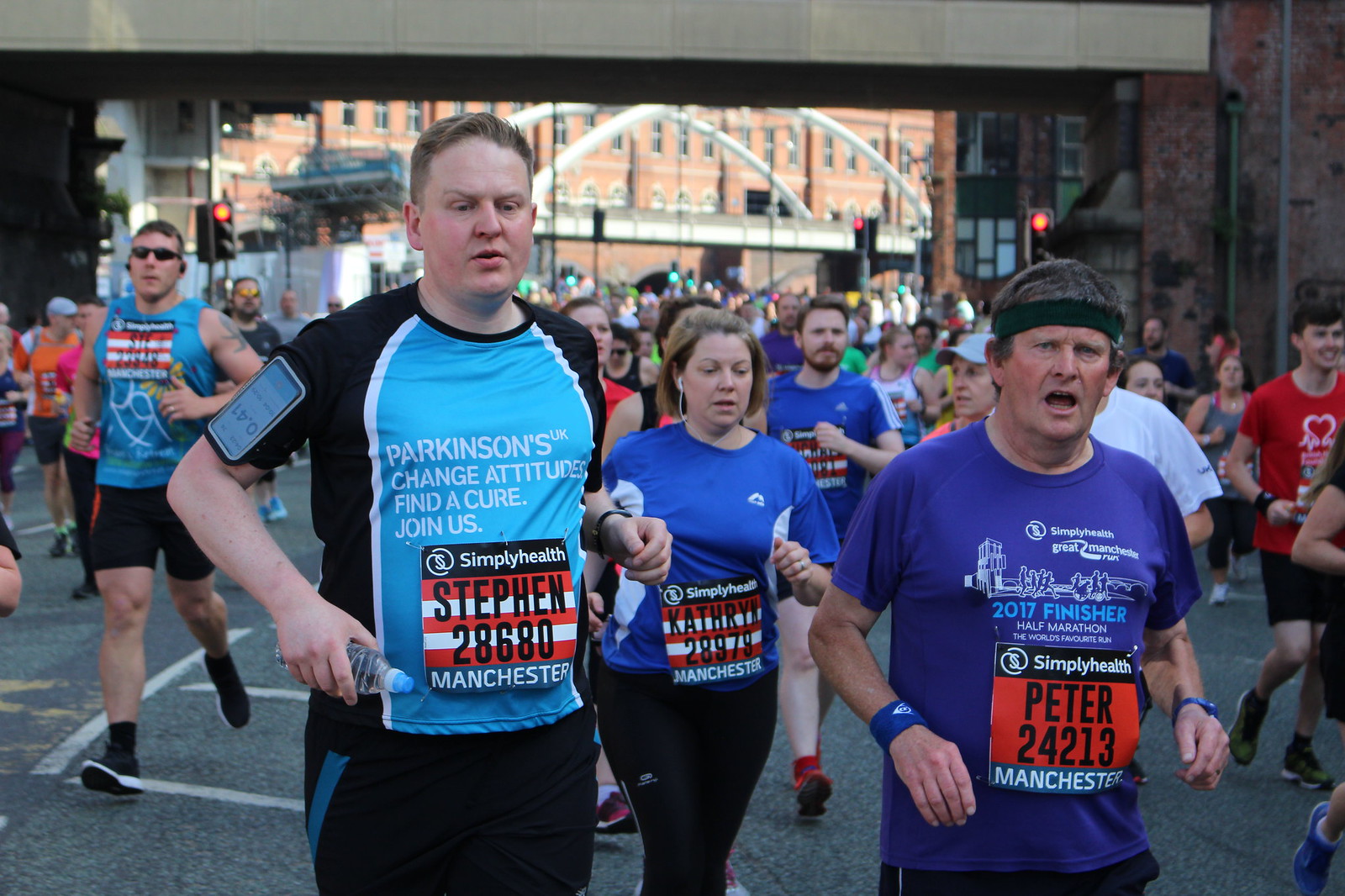In this outdoor marathon event, hundreds of participants fill the scene, some adorned in vibrant colors including peach, black, white, yellow, green, red, purple, light blue, gray, and orange. The front of the image prominently features three runners. On the left, Stephen sports a shirt with a light blue center and black sleeves and shorts. His shirt bears the message "Parkinson's: Change Attitudes, Find a Cure, Join Us," and his race bib reads "Stephen 28680 Manchester." Stephen also has a phone strapped to his sleeve. In the middle, Catherine wears a blue shirt with white accents and black leggings, her race bib reading "Catherine 28978 Manchester." To the right, Peter dons a purplish-blue shirt, a black headband, and his race bib says "Peter 24213 Manchester." Behind them, rows of runners are visible beneath a sky lined with buildings and a bridge, with stoplights framing the street. The runners appear to be part of a large community event, united in motion and purpose.